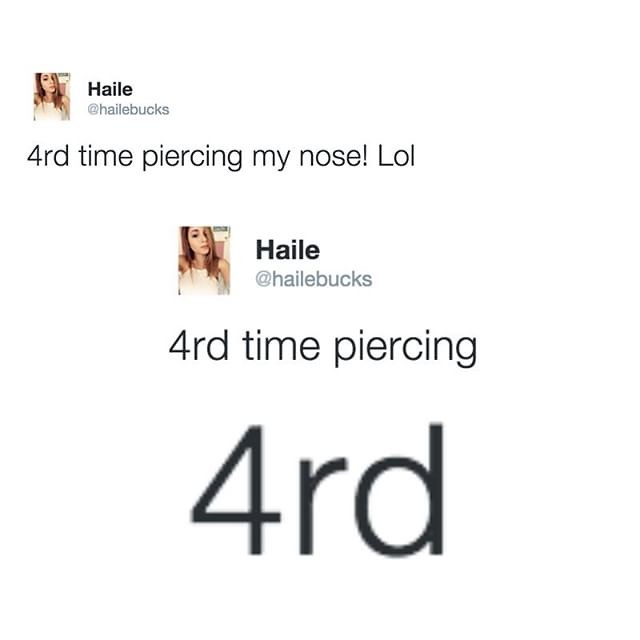The image is a color portrait-format screenshot from a social media platform. The backdrop is a clean white interface, suggesting it could be a tweet or an Instagram post. At the top left corner, there is a small profile picture of a woman with brown hair, wearing a white top, looking directly at the camera. Accompanying the profile picture is the name "Haile" (H-A-I-L-E) in black text, with the handle "@HaileBooksBox" in gray text below it.

Centered prominently in the image is her post, which reads: "Ford Time Piercing My Nose LOL" with a mix of black and gray text, emphasizing informal humor. Below this post, the message "Ford Time Piercing" is repeated, highlighting the phrase "4RD" in noticeable black text, playfully referring to "4th" as "Ford." The same profile picture and name are repeated above and below this post, consistent throughout the image. The overall background remains white, keeping the viewer’s focus on the textual content and the profile details.